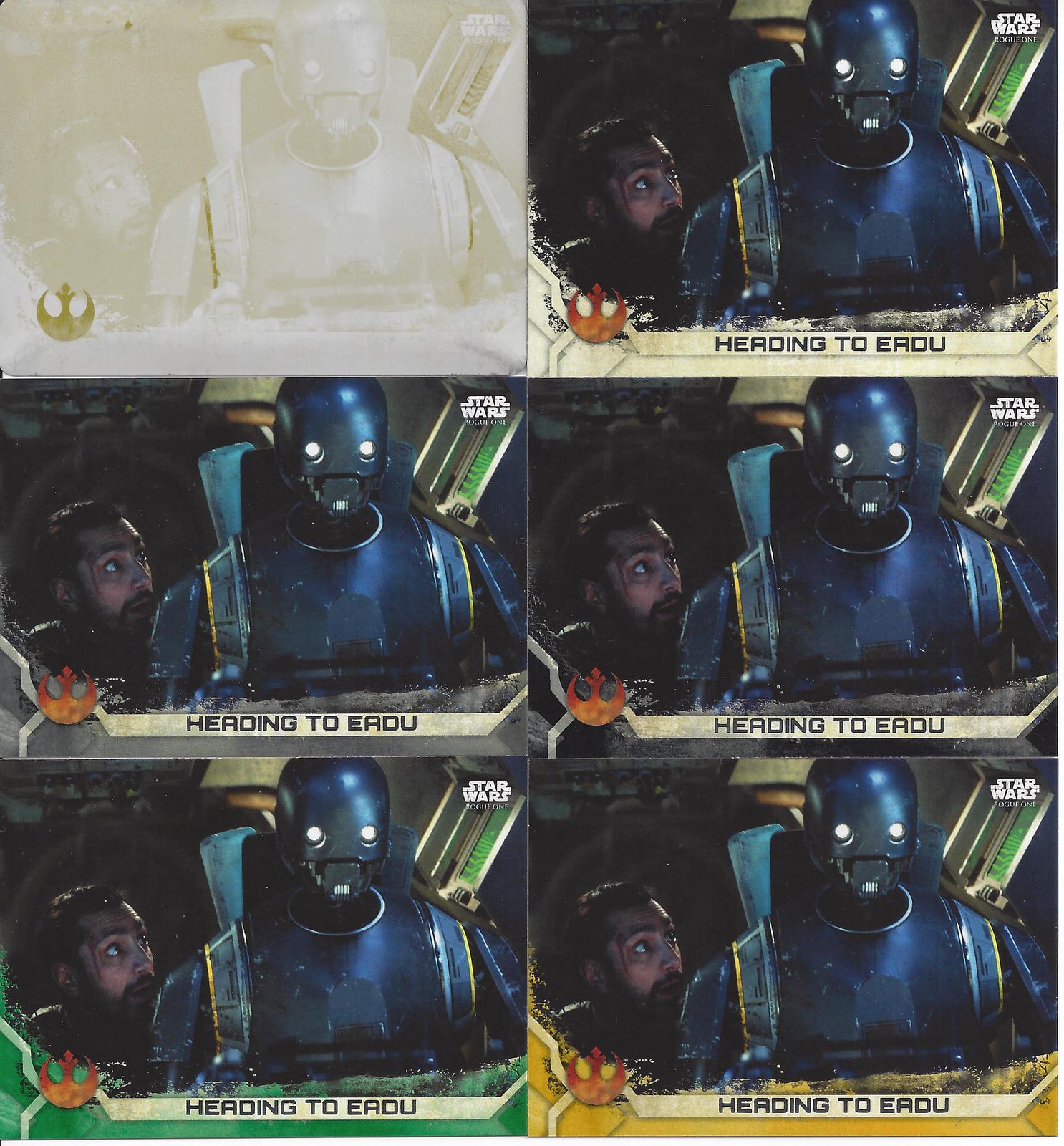This image showcases six Star Wars Rogue One trading cards, each featuring the same scene with a robot and a man. The man, with dark black hair, a mustache, beard, and brown skin, is peeking up from the side of the frame, a streak of blood on his face. He seems to be observing the robot, who has lit-up eyes and appears to be seated in a pilot position. The top left card has a distinct appearance, with a shadow cast over it, making it yellowish-brown. The top right card displays a Star Wars Rogue One title. Each card's bottom banner has the text "Heading to" with the Rebel Alliance logo, differing in color: the bottom banners vary in yellow, gray, dark gray, green, and a darker yellow, indicating different parallels, possibly signifying different levels of rarity. The top left card seems to be a special "press proof" version, lighter and slightly washed out in comparison to the others.